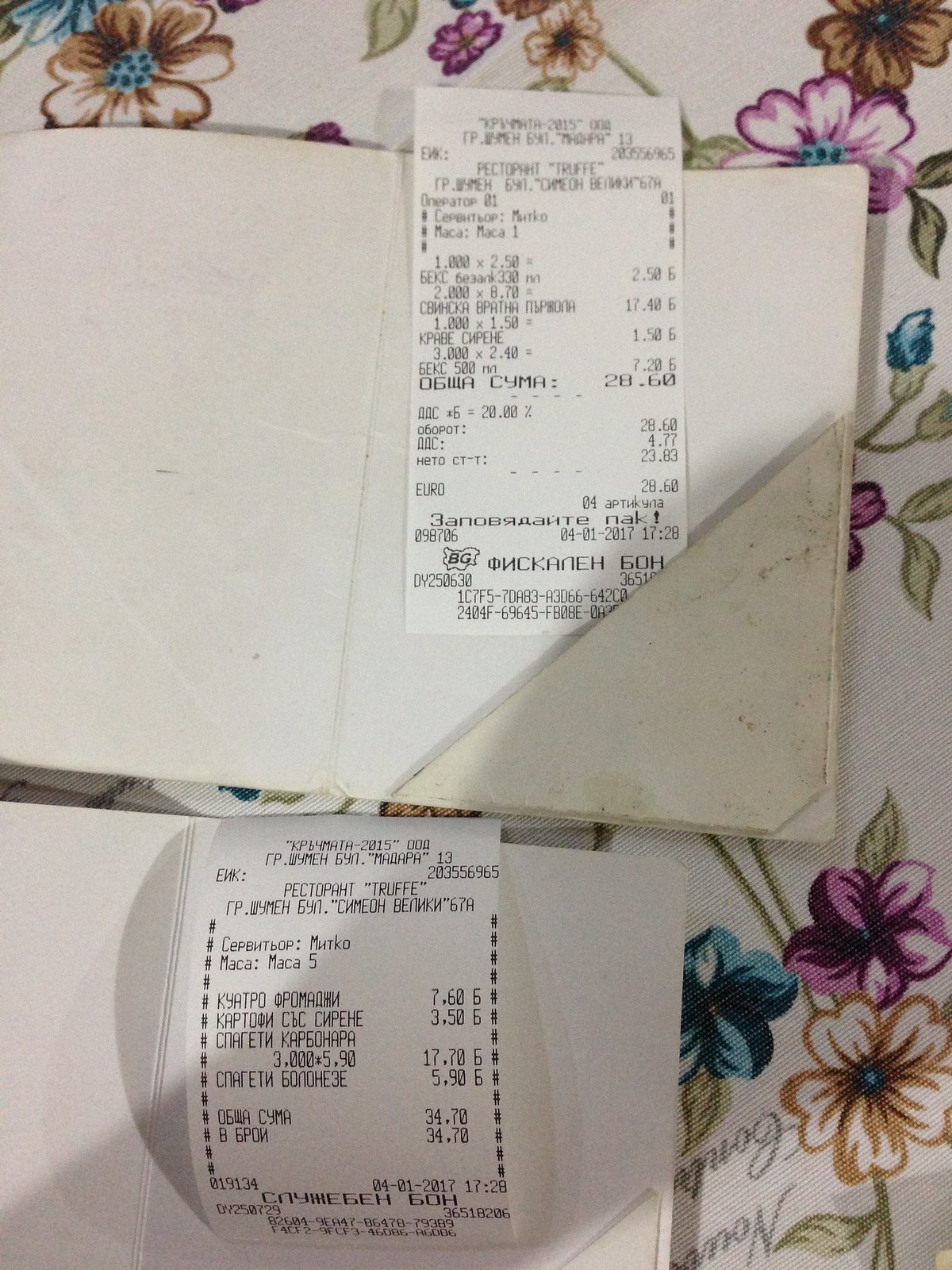The image features two receipts, each nestled in a dedicated cardboard booklet designed specifically for holding them. These booklets include a holder mechanism on the right corner, ensuring the receipts stay securely in place. 

The booklets are arranged one above the other, laid flat on a table adorned with a floral-patterned tablecloth. The photograph is taken from a top-down perspective, offering a clear view of the setup.

Though the details on the receipts are somewhat difficult to discern, it is apparent that the total amount on the top receipt reads $28.60, while the bottom receipt shows a total of $34.70. The overall presentation suggests an organized and tidy record-keeping system.